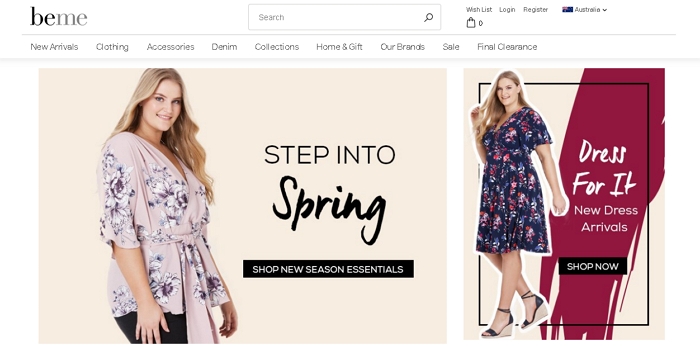**Website Screenshot Description: E-commerce Clothing Store "BeMe"**

In this detailed screenshot of a clothing retail website named "BeMe," the logo is prominently displayed in the upper left corner. The logo, "BeMe," is styled with "B-E" in bold and "M-E" in regular font, all as a single word. Directly to the right of the logo, there is a search bar featuring a placeholder text that reads "search" accompanied by a magnifying glass icon.

Adjacent to the search bar are quick access options labeled "Wishlist," "Login," "Register," and the country indicator "Australia."

Beneath the top navigation bar, a secondary menu provides selectable categories, including: 

- New Arrivals
- Clothing
- Accessories
- Denim
- Collections
- Home and Gift
- Our Brands
- Sale
- Final Clearance

Below this navigation menu, two large promotional images dominate the screen. Both images showcase the same young woman with long, wavy blonde hair flowing past her shoulders.

- The image on the left features the woman dressed in a pink top adorned with a white and purple floral pattern, paired with black pants. An overlay on a tan background reads, "Step into Spring, Shop New Seasonal Essentials."
  
- In the image on the right, set against a tan background with a navy paint smear effect, the same woman is shown wearing a vibrant blue, red, and white floral dress. The text overlay here reads, "Dress for It, New Dress Arrivals, Shop Now."

Both promotional sections invite users to explore and shop the latest seasonal and dress arrivals.